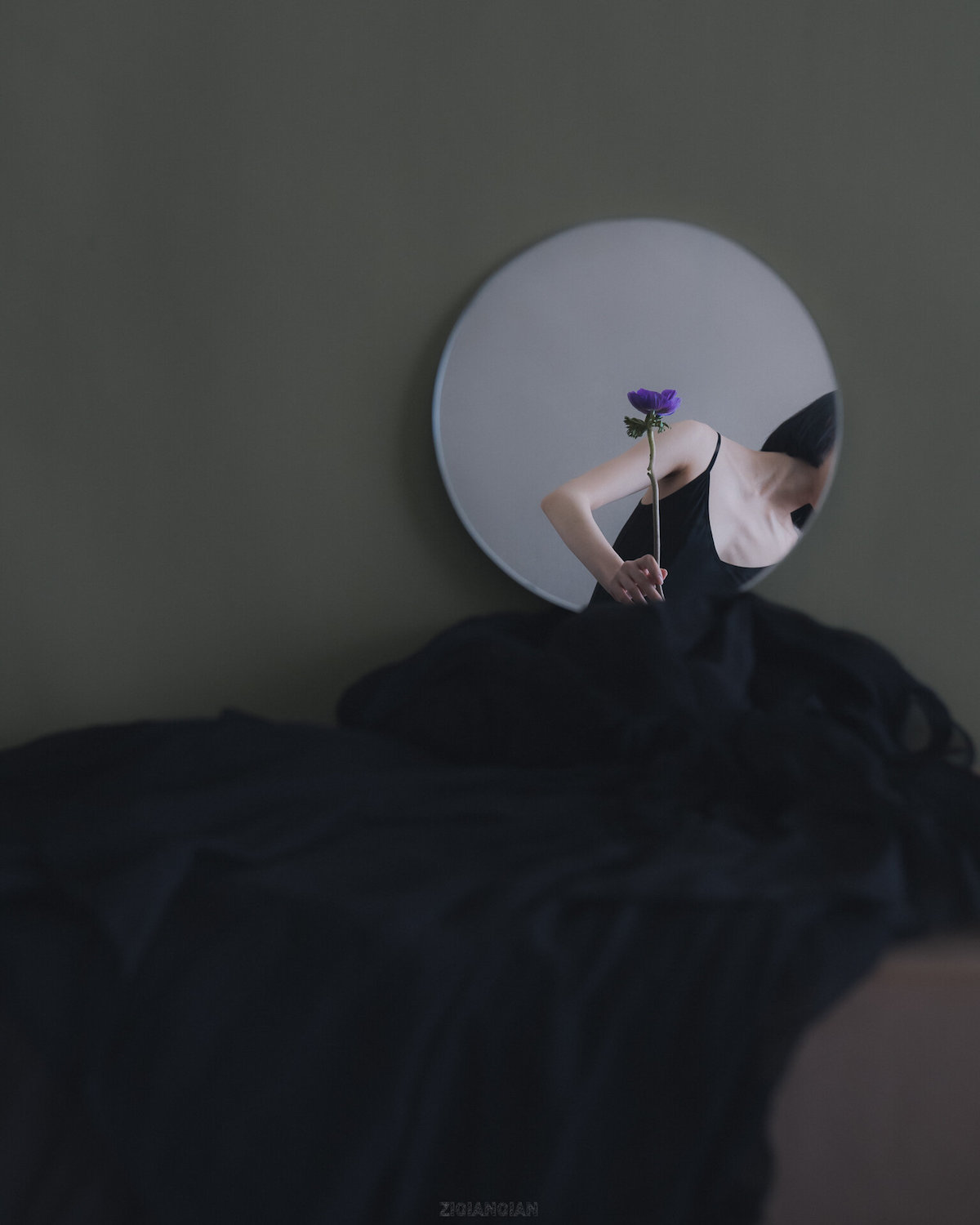The image depicts a woman in a striking and voluminous black gown with spaghetti straps and a tight-fitting bodice, prominently showcasing her thin frame and pronounced collarbones. She holds a purple flower in her right hand, with her arm elegantly bent. Her short black hair, which doesn’t reach her shoulders, is seen as her head is turned away, obscuring her face. The central focus of the composition is a large, round mirror with a silver edge. The woman leans far to the right, and her reflection in the mirror captures her chest and the black gown while her head remains outside the mirror's view. Below the mirror, a substantial amount of dark cloth is bunched together, spilling off towards the left. The background is a medium gray, with a purplish-gray area in the bottom right adding to the muted yet sophisticated color palette. The positioning of both the woman and the mirror creates an intriguing interaction between the reflection and the actual figure.